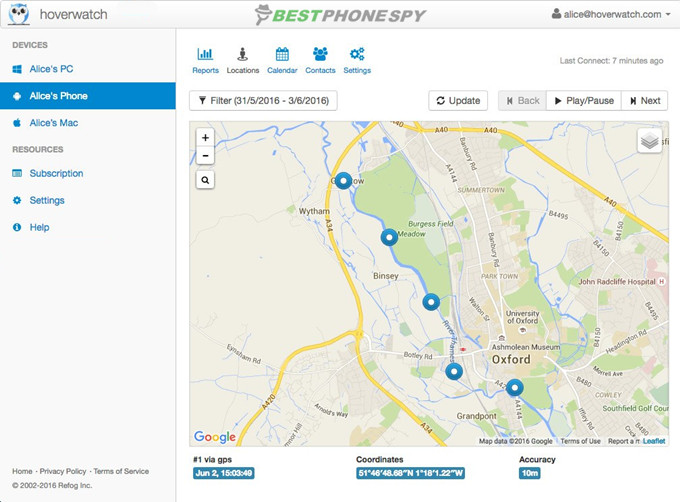This image depicts an interface from the application "Best Phone Spy," which allows users to track the location of certain devices they own. The primary interface displays a map around the Oxford area, marked with multiple lines indicating the tracked movements of various items. Specifically, the user is monitoring three devices: Alice's PC, Alice’s phone, and Alice's Mac. 

At the top of the interface, the user can navigate through tabs labeled Reports, Locations, Calendar, Contacts, and Settings. This particular view showcases the locations of the devices filtered by date, specifically from May 31st, 2016 to June 3rd, 2016. Coordinated spots on the map denote the precise locations of the tracked devices with an accuracy of 10 meters, and the most recent data point is from June 2nd at 15:03:49. 

On the left side of the screen, additional navigation options include Subscription, Settings, and Help, suggesting that the application operates on a paid subscription model. The email registered to this account is alice@hoverwatch.com. The map itself is sourced from Google Maps, as indicated by the Google logo at the bottom of the interface. Users have the ability to zoom in, zoom out, and search for more detailed information directly within the application.